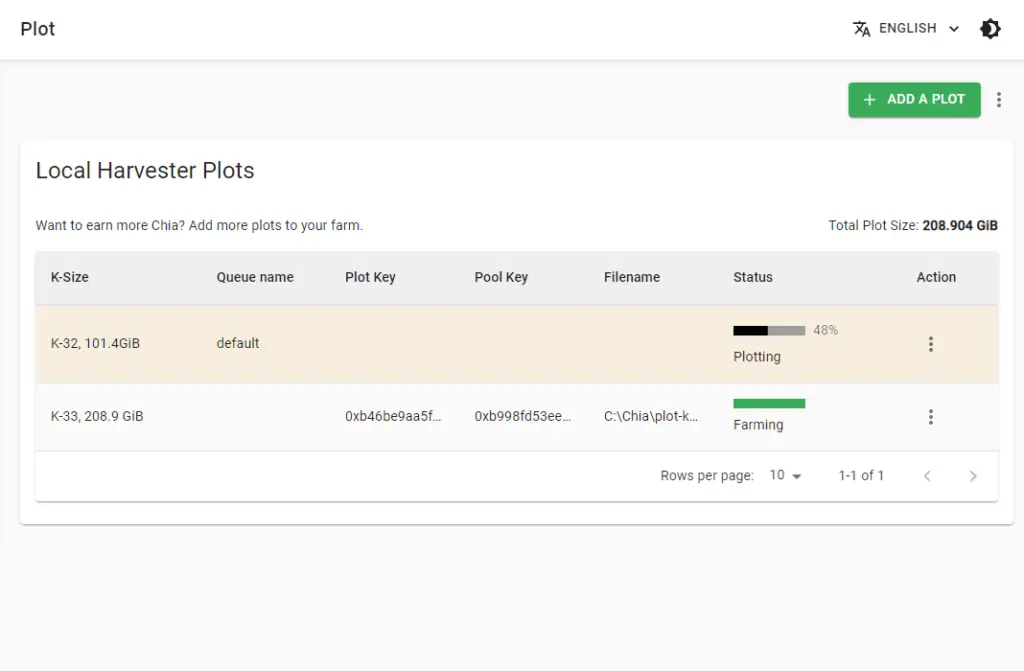The image has a distinct white border at the top, featuring the word "Plot" in black text on the upper left. On the far right of this border, there is a drop-down menu labeled "English," accompanied by a black gear icon to its right. Beneath this, there is a rectangular section with a gray border at the top and a white background in the middle. 

At the far right of the gray border, a green rectangular button labeled "+ Add a Plot" is visible. Within the white portion of this rectangle, the upper left corner contains the text "Local Harvester Plots." On the far right, there is a message reading, "Want to earn more? Add more plots to your farm."

Further down, there is a gray line displaying the headings: "Case Size," "Queue Name," "Plot Key," "Pool Key," "File Name," "Status," and "Action." Below this, a beige line indicates the details: "Default" and "Plotting," which appears to be around 45% complete.

Underneath this section, another gray bar informs you that you are currently farming, with a green line present above this message. Finally, at the bottom of the image, there is an option showing that you have selected "10 rows per page" for the displayed rows.